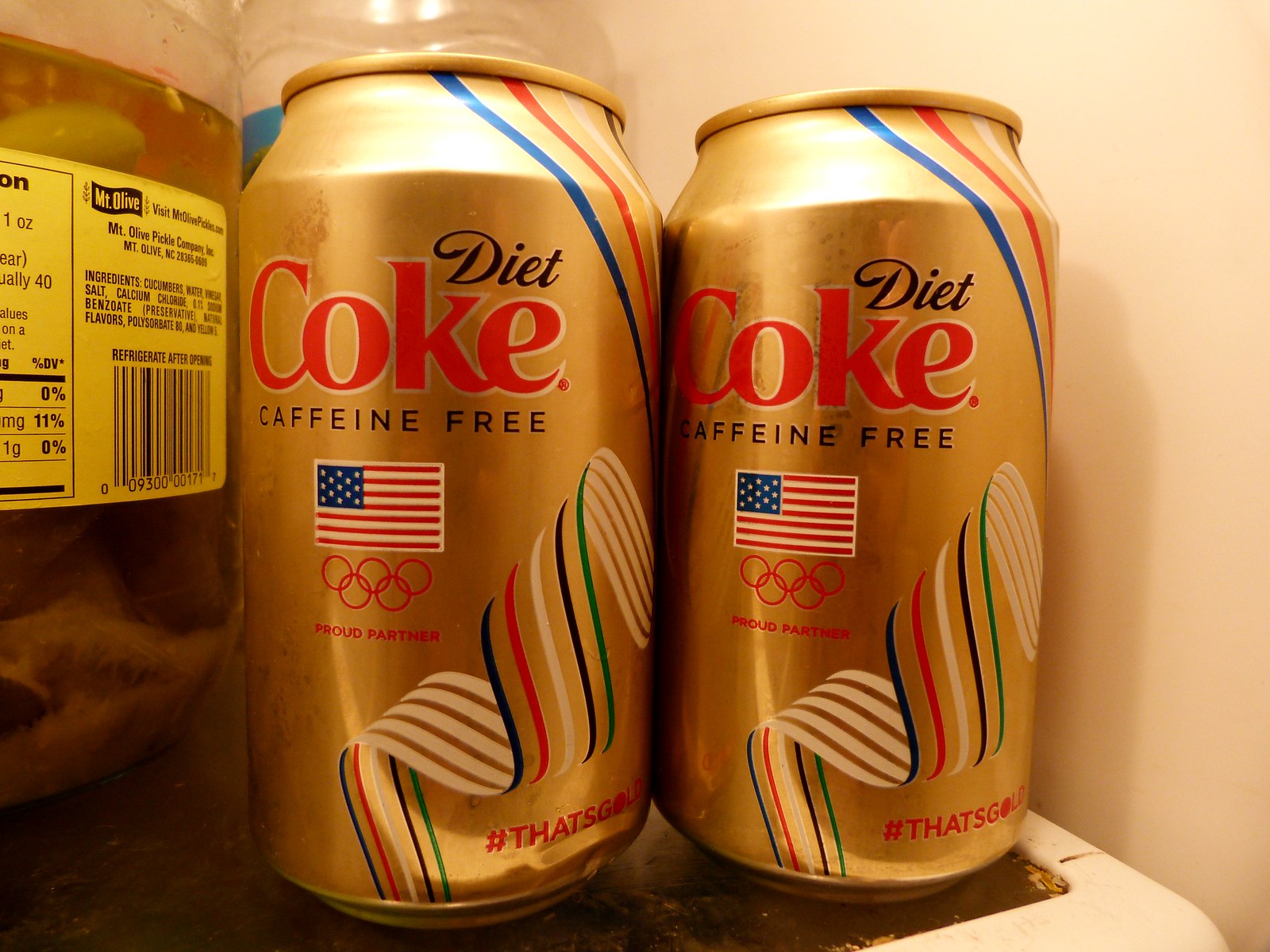This photograph captures a close-up of two limited edition Diet Coke cans inside a refrigerator. The cans are adorned in a striking gold color, accented with red, white, and blue stripes and an American flag, making it evident that they are themed for a special occasion. These cans appear to be part of a promotional campaign supporting Team USA for the Olympics. Beneath the American flag on the cans, the iconic Olympic rings are displayed, reinforcing the connection to the international sporting event. Additionally, the cans feature a ribbon-like design in the five Olympic colors: red, white, blue, black, and green. Each can is labeled "caffeine-free" and includes a hashtag at the bottom in bold red letters, which reads "That's Gold," likely a nod to the pursuit of gold medals in the Olympics. This patriotic and celebratory design ties together the gold medal theme with the gold color of the cans, creating a cohesive and eye-catching tribute to the Olympic Games.